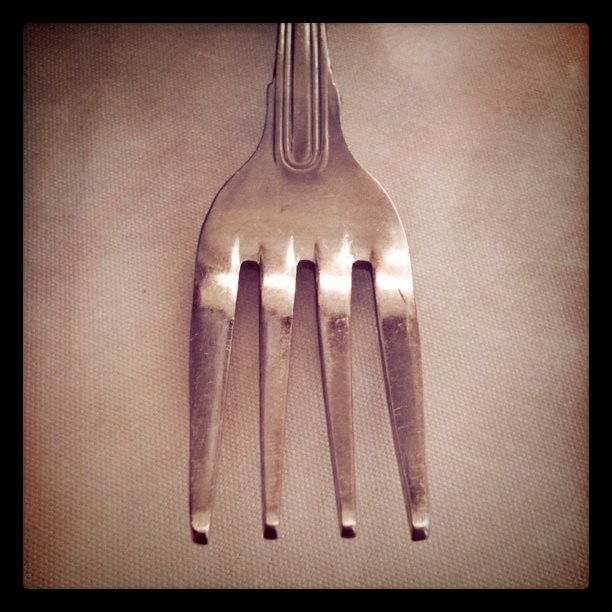This image captures a meticulously detailed, close-up view of the head of a vintage fork. The fork, a somewhat tarnished stainless steel utensil displaying signs of age and wear, sits on a plain white surface that appears to be fabric. The photo is tinted with a reddish-brown sepia tone, lending an antique feel. The focus is on the head of the fork, featuring four wide, blunt tines that are not sharp, suggesting it is designed for eating foods like salads or meats. The tines exhibit noticeable scratches and a patina, indicating their long usage. Light reflections on the metal reveal the dull sheen of a fork that has seen many years of service. The handle of the fork is partially visible, adorned with a simple inset design and showing significant wear, further emphasizing its vintage nature. No other objects are present in the frame, directing full attention to the intricate details and textures of the fork itself.